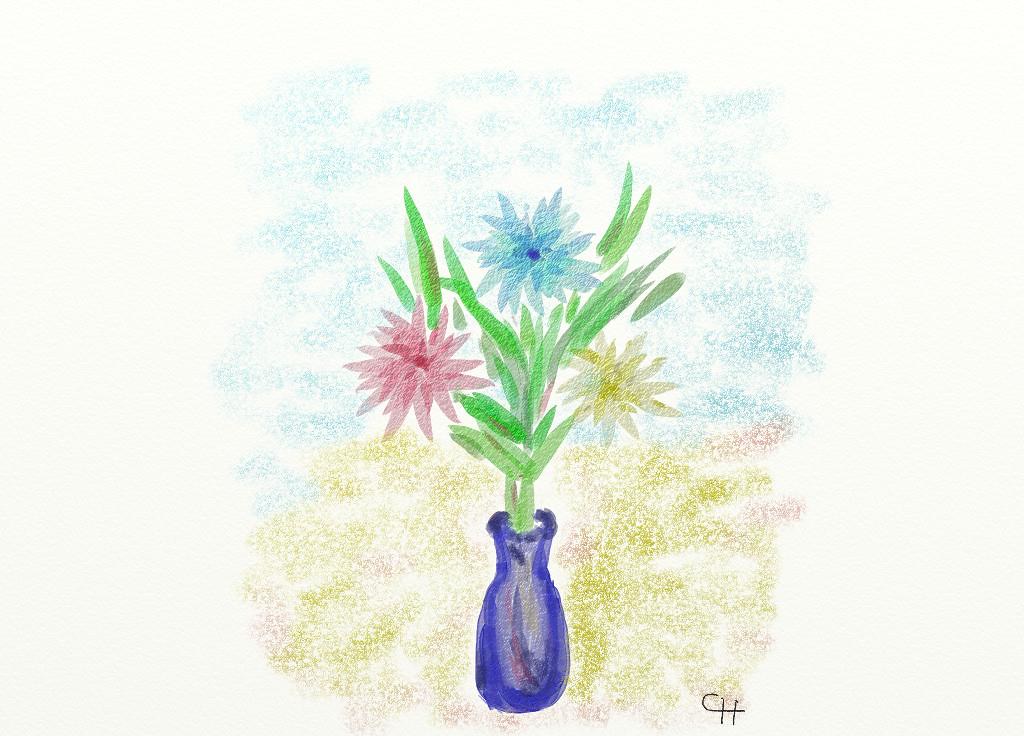This watercolor painting features a vividly detailed flower vase, signed "CH" in stylized black lettering in the bottom right corner. The vase itself displays a rich purple hue with intricate shadings of gray, enhancing its depth and texture. Emerging from the vase, the flowers are arranged in a triangular composition. At the center, delicate pink blossoms capture the viewer’s attention, transitioning to blue flowers at the top and mustard yellow blooms on the right-hand side. Surrounding the flowers, medium green foliage adds a touch of natural greenery. The background is a soothing blue, blending effortlessly into green hues at the bottom, offering an abstract sense of depth without indicating a specific setting. The painter's technique combines the light, fluid qualities of watercolor with thoughtfully drawn outlines, resulting in a harmonious and visually appealing piece.